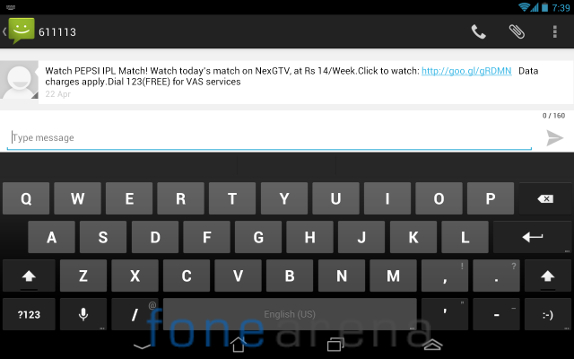The image depicts a webpage displayed on a computer screen with an on-screen keyboard visible. The on-screen keyboard is primarily black with gray keys, creating a stark contrast. The keyboard features a smiley face in a green square, followed by the number "611113." To the far right of the keyboard are icons of a traditional hook phone, a paperclip, and three vertical dots stacked one above the other.

Above these elements, the status bar displays typical indicators: a Wi-Fi signal strength icon, a phone battery strength symbol, and a timestamp showing "7:39."

Beneath the status bar, white text stands out against a dark background. The text reads: "Watch Pepsi ILP MATCH! Watch today's match on NextGTV at RS14/week. Click to watch" with an accompanying link and the notice "Data charges apply." Additionally, there's an instruction to "Dial 123 free for VAS services."

Below this text box is an input area where users can type their messages. At the bottom of the screen, navigation icons are visible, including a downward arrow, a home button, a screen up button, page up and page down buttons, or a button to make the page smaller.

Faintly faded into the background is the text "FONEarena," with "FONE" in blue and "arena" in gray, overlaid on the on-screen keyboard.